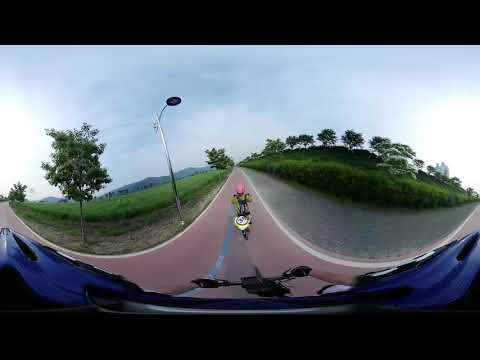The image appears to be a distorted, panoramic photograph taken from the perspective of a GoPro mounted on someone's helmet, giving it a fisheye effect. The foreground shows the handlebars of a blue motorcycle, with the rider's white arms clad in black gloves gripping them. Ahead, another motorcyclist can be seen from the back, wearing a gray helmet and orange clothing with a white backpack. The rear of their bike features a yellow section with a number 36 sticker. Both riders are traveling down a reddish-brown paved road, devoid of line markings, bordered by lush green grass and scattered trees. To the left of the road, there's a single streetlight and a field, while the right side shows a cleared cement area leading up to a hill with trees. In the distance, light gray mountains frame the horizon against a clear blue sky.